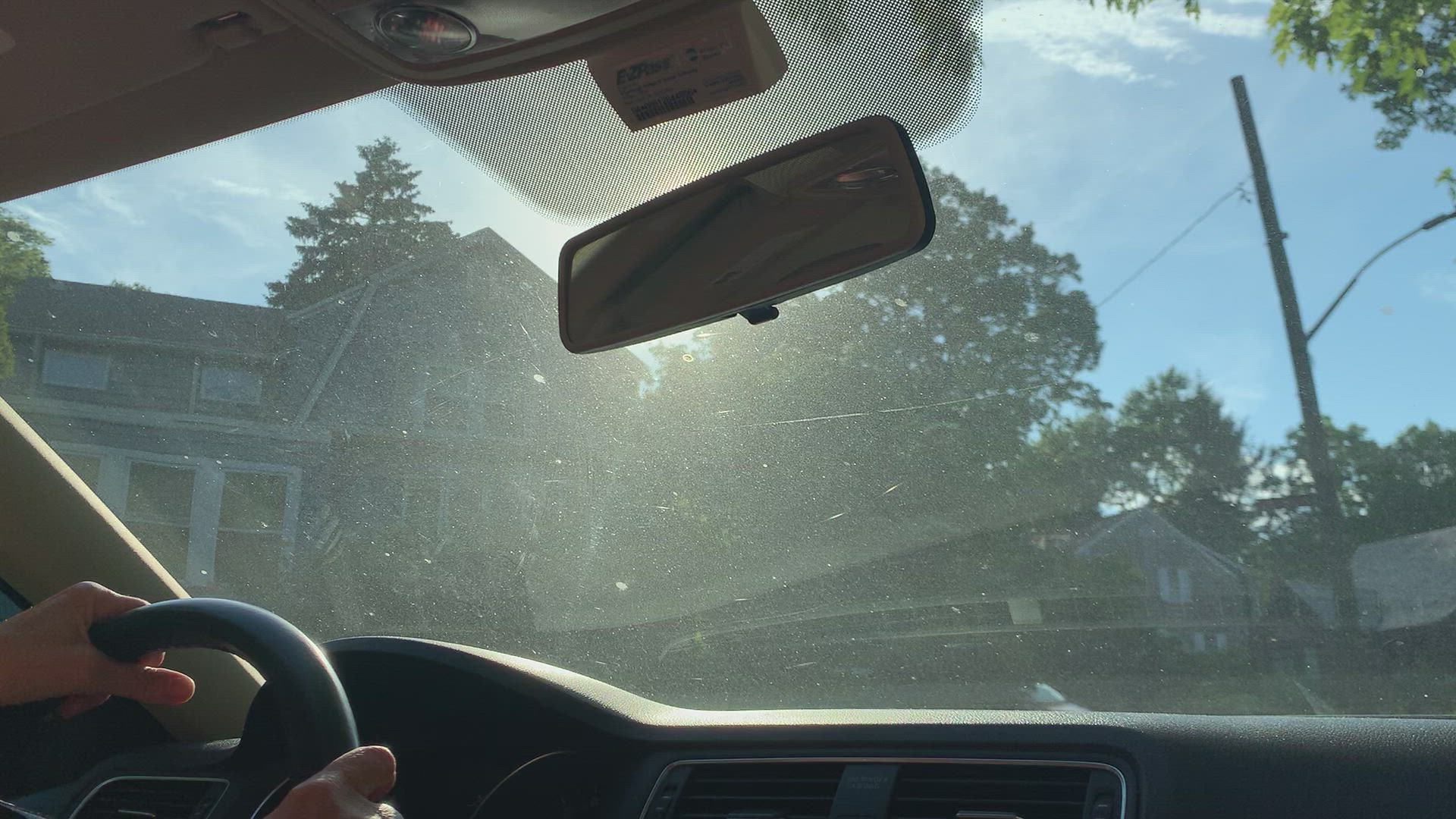Captured from the passenger side of a vehicle, this photo offers a glimpse into a typical suburban drive. The interior showcases a black dashboard with partially visible fan vents and a rear-view mirror that creates a mild sun glare, refracting the bright midday light. The driver’s hands are seen gripping the steering wheel, suggesting a steady focus on the road ahead. Through the windshield, a serene residential neighborhood unfolds, framed by tall, leafy trees against a vivid blue sky. Two-story houses align the street, hinting at a well-maintained and pleasant community. The sun’s rays, gently blocked by the rear-view mirror, cast soft beams, adding a warm glow to the scene.